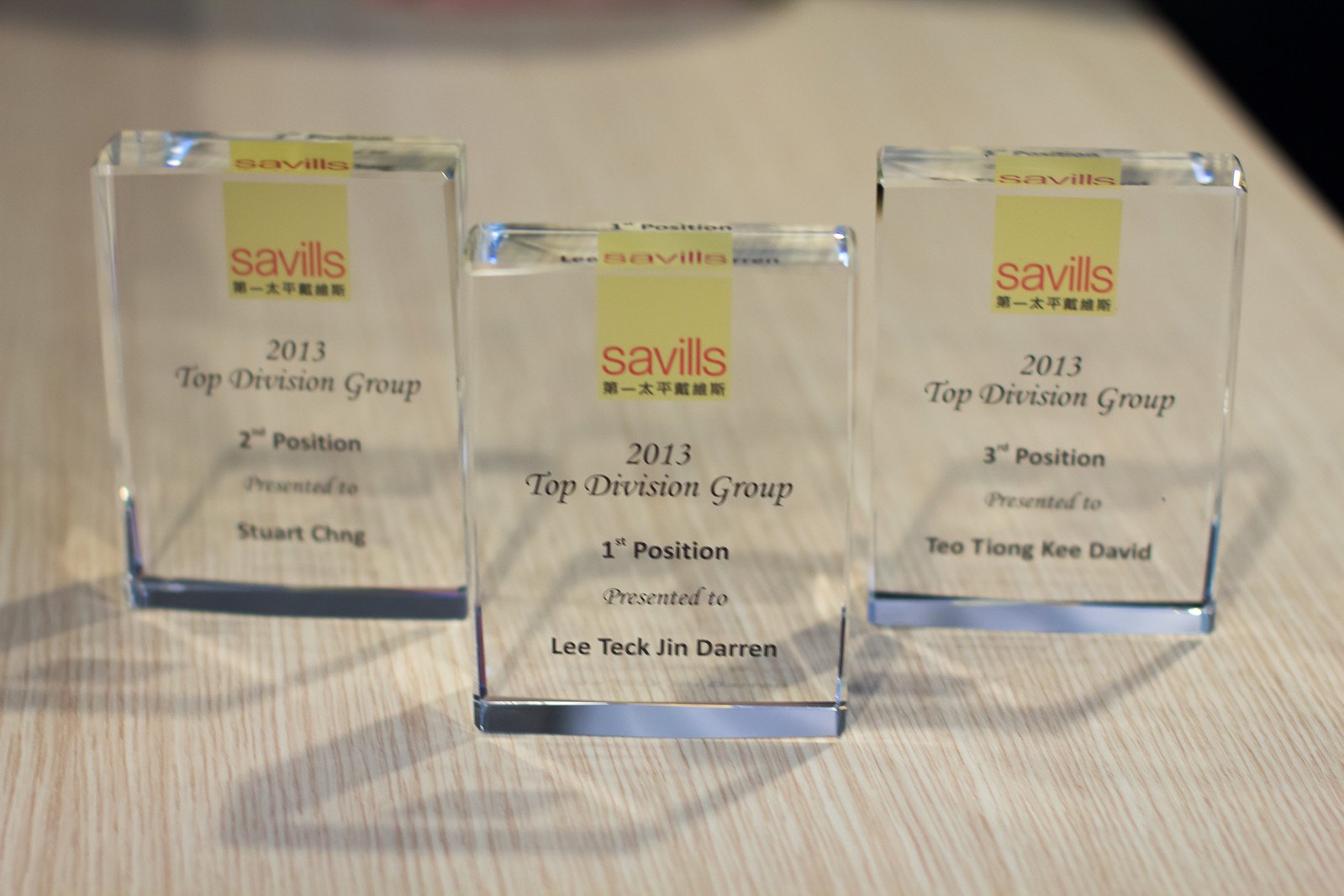The image showcases three elegant, translucent glass awards meticulously arranged on a light tan wooden table with subtle white ridging. These awards are positioned in a pyramid-like formation, with the central award slightly ahead of the two flanking it. Each award features a prominent yellow box at its upper center, displaying the word "Savills" in bold red font, followed by additional text in a Chinese dialect and the phrase "2013 Top Division Group" in black. The awards are distinguishable by the inscriptions at their lower half: the middle award honors Li-Tech Jin Darin with the first position, the left award recognizes Stuart Cheng with the second position, and the right award acknowledges Teo Tiong Kee David with the third position. Each award is securely mounted on a sleek, half-inch silver base, enhancing their refined and fragile appearance.